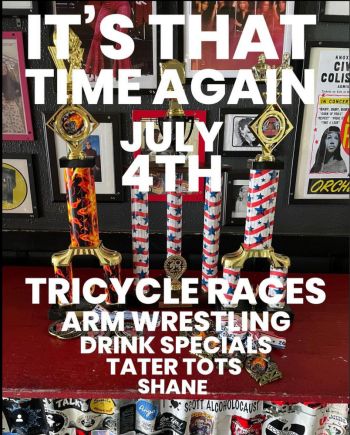This horizontal advertisement poster showcases an event with layered details. Prominently displayed in bold white letters at the top is the phrase "It's that time again," followed by "July 4th" centered beneath it. Below, the poster lists activities and offers: "Tricycle Races," "Arm Wrestling," "Drink Specials," "Tater Tots," and the name "Shane."

The background features a collection of objects and imagery. A red shelf sits in the middle of the scene, adorned with three or four golden trophies. The wall behind this shelf is grey and slightly textured, holding an array of framed pictures and artwork. Below the shelf, white designs appear to mimic newspaper clippings pasted to the wall. Lining the bottom of the image are what seem to be cans of beer.

The photograph employs a rich color palette including white, gold, yellow, orange, dark red, black, light blue, and dark blue. The setting seems to be indoors, though the time of day remains indeterminate.